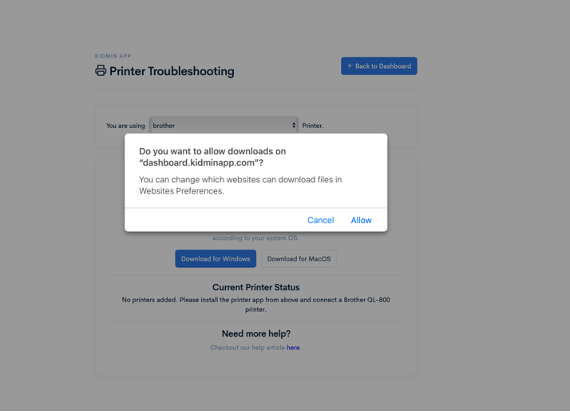The image captures a digital screen displaying a printer troubleshooting interface. The header "Printer Troubleshooting" is prominently shown in black text on a gray background. To the right of the header is a blue button with white text.

Dominating the center of the screen is a large white pop-up text box with a notification that reads: "Do you want to allow downloads on dashboard.kidnap.com? You can change which websites can download files in Website preferences." Beneath the notification, there are two buttons: a blue "Allow" button and a gray "Cancel" button, both with white text.

Below this pop-up, the screen displays a section titled "Compact Printer Status" with additional text reading "Need more help?" accompanied by more blue text below.

In the top left corner of the screen, a small black printer icon is visible, providing a visual cue related to the printer troubleshooting context.